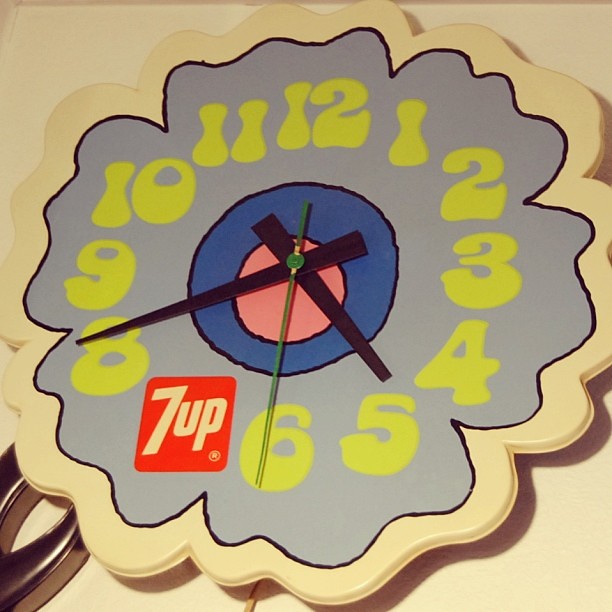This color photograph captures a distinctive flower-shaped analog wall clock set against a light beige background. The clock features a playful, cartoonish design with scalloped, roughly-edged petals. The outer part of the clock face is a light lavender color, outlined in thin black. In the center lies a medium blue circle encircling a solid pink circle. Vibrant neon yellow numbers, rendered in a cartoony font, surround the clock face. A notable detail is the 7UP logo replacing the number 7, presented in red and white. The black hour and minute hands indicate the time as 20 minutes to 5, while a green second hand points at the number six.